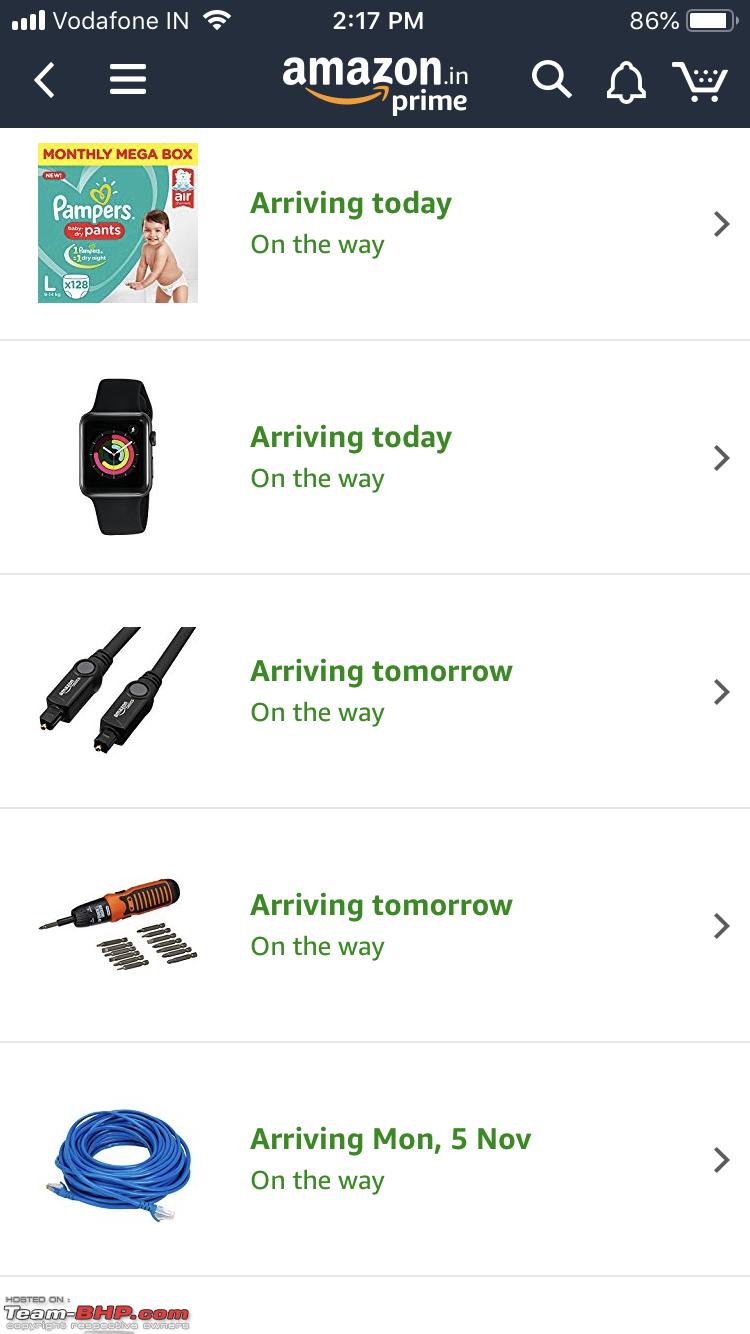This screenshot from an Amazon India app on a smartphone displays detailed information about an order. The dark grey top border features the Amazon logo in white, with 'dot IN' in small letters next to it and the iconic smile logo underneath, followed by the Prime logo. In the upper left corner, the wireless connection icon indicates Vodafone India (V-O-D-A-F-O-N-E-I-N), while to the right, the Wi-Fi icon is visible. The time, centered just above the Amazon logo, reads 2:17 p.m. On the upper right corner, the battery icon shows an 86% charge.

Below this section, the background turns white, presenting details of five items ordered. Each item is accompanied by its image on the left and a status update in green on the right, stating "Arriving today" and "On the way" for each product. The ordered items include:

1. A package of Pampers.
2. A smart watch.
3. Two USB cables.
4. An unidentified tool-like item.
5. A notably long blue cable.

This comprehensive layout reflects the user's active order list with clear visual and textual information.